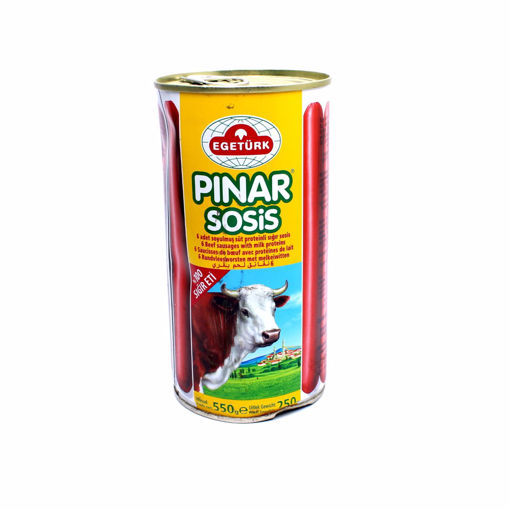The image features a tall, unopened can positioned against a completely white background, typical of a product photo for a supermarket website. The cylindrical can has a pop-top lid and prominently displays the brand name "EGRATURK" near the top, with "Pinar Sosis" in bold white letters across the middle. The can's label is primarily yellow with red accents on the sides, possibly depicting sausage links or meat sticks. A stylized image of a cow with horns is situated on the bottom half of the can, set against a scenic backdrop of a grassy meadow with a blue sky and small buildings in the far distance. The detailed artistic depiction of the cow, along with the overall design, suggests that the product inside could be beef sausages. The can shows slight dents on the upper left and bottom.